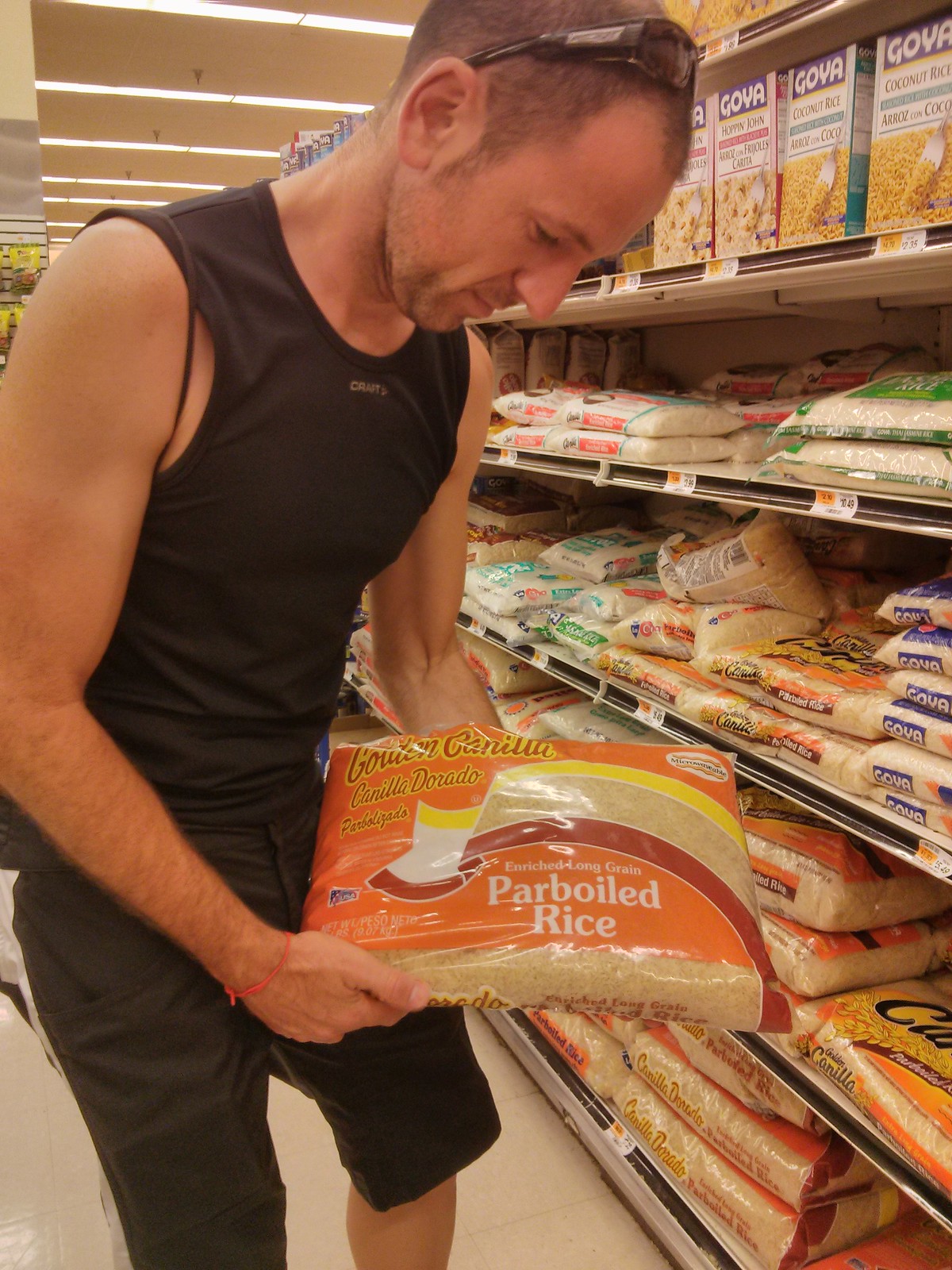This vertical, color photograph depicts a young man, likely in his 30s, with very short hair and medium skin, shopping in a grocery store. He sports black sunglasses perched on his forehead, a black tank top, and black shorts that fall to his knees. An apricot or reddish-pink wristband adorns his wrist. The man is focused on a large bag of parboiled rice labeled "Golden Canela" in white text against an orange background, with additional brown and yellow stripes. Shelves filled with various brands of rice including Goya, as well as other grains and boxed foodstuffs, stretch from the floor to the beige ceiling, which is illuminated by horizontal fluorescent lights. The tan floor grounds the scene, emphasizing the array of products in the bustling retail environment.